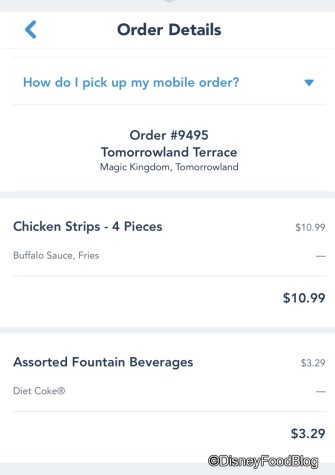This image is a screenshot taken in portrait mode from a phone, displaying an order receipt on a Disney food blog site. At the very top, the image features a gray stripe that extends across the upper left and upper right corners. On the next row, there is a blue back arrow on the left, and at the center, the phrase "Order Details" is prominently displayed in bold font. 

Below this, another row appears, instructing users on "How do I pick up my mobile order?" with a small blue downward-facing triangle at the end of the line, indicating a dropdown menu.

The next section lists "Order #9495" for "Tomorrowland Terrace" located in "Magic Kingdom Tomorrowland." A gray stripe appears beneath this information. 

Subsequently, the order details are presented, starting with:
- **Chicken Strips (4 pieces) - $10.99**, including buffalo sauce and fries. 
Another gray stripe follows underneath.

Next, the beverage order is displayed:
- **Assorted Fountain Beverages - $3.29**, specifying a Diet Coke. The price $3.29 is also highlighted in bold.

In the bottom right corner of the screenshot, the source "Disney Food Blog" is noted, signifying that this receipt visualization comes from their website. The overall image illustrates the receipt of a mobile order placed for a meal at Tomorrowland Terrace, part of the Disney Food Blog's demonstration of the ordering process.